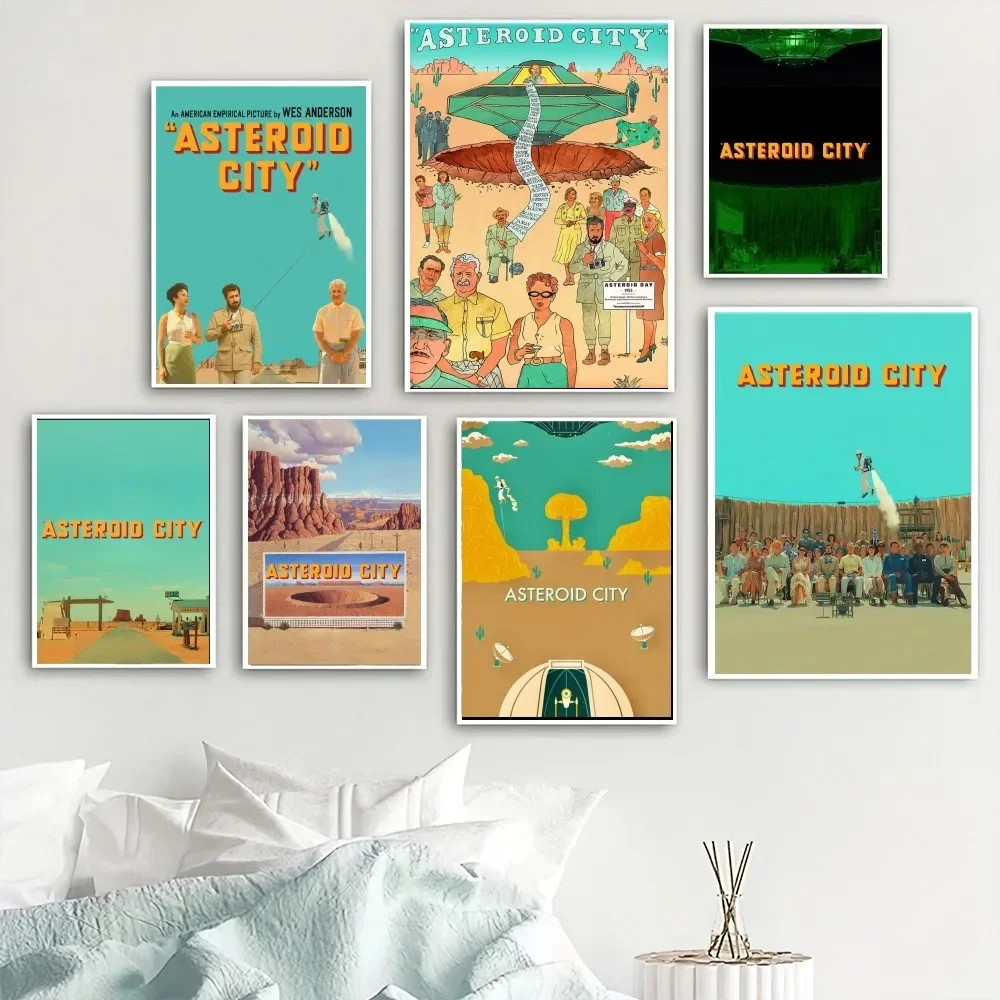The image features a bedroom with a wall adorned by a detailed montage of seven framed posters related to the film "Asteroid City." The arrangement includes three at the top, four at the bottom, with the largest poster positioned in the middle of the top row. This central upper poster is an illustrated depiction of characters from the movie, while the lower right poster is an actual group photograph of the cast. There are two smaller posters on the left and one on the right. The lower left and third from the left on the bottom showcase more austere designs.

In the room, an unmade bed with white sheets, a white blanket, four white pillows, and a teal-colored sheet occupies the left side. Adjacent to the bed, on the right, stands a small white table holding a glass with chopsticks, possibly paint brushes, and a diffuser. The rightmost poster with gold lettering reads "Asteroid City" and depicts three people either standing or sitting in a desert setting. Another poster shows a spaceship with people fleeing from it. The varied posters bring a vibrant, cinematic ambiance to the otherwise simple bedroom setup.